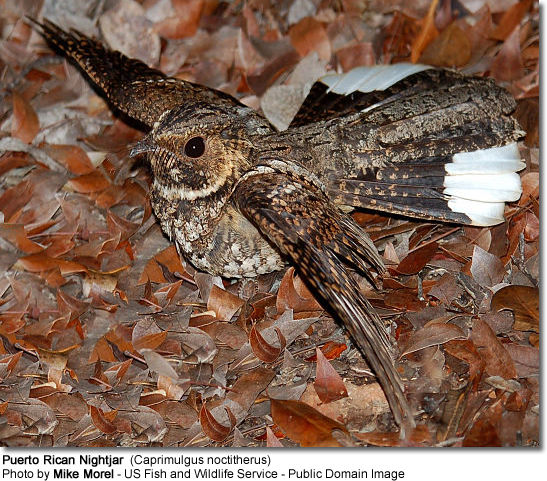This detailed photograph, taken by Mike Morrell of the US Fish and Wildlife Service and available in the public domain, captures the elusive Puerto Rican Nightjar (Caprimulgus noctitherus). The bird, well-camouflaged within a bed of dark orange and brown leaf litter, displays its cryptic plumage. Its predominantly brown feathers feature intricate speckling on the stomach, blending seamlessly with the forest floor. A distinctive characteristic is its white-tipped tail, contrasting with the rest of its brown body. The bird's left eye, small and black, is visible and adds a sharp contrast to its subdued feather coloring. With wings outstretched, the Puerto Rican Nightjar's brown beak and unique plumage details come into clear view, making this image a valuable documentation of a rare and often hidden species.